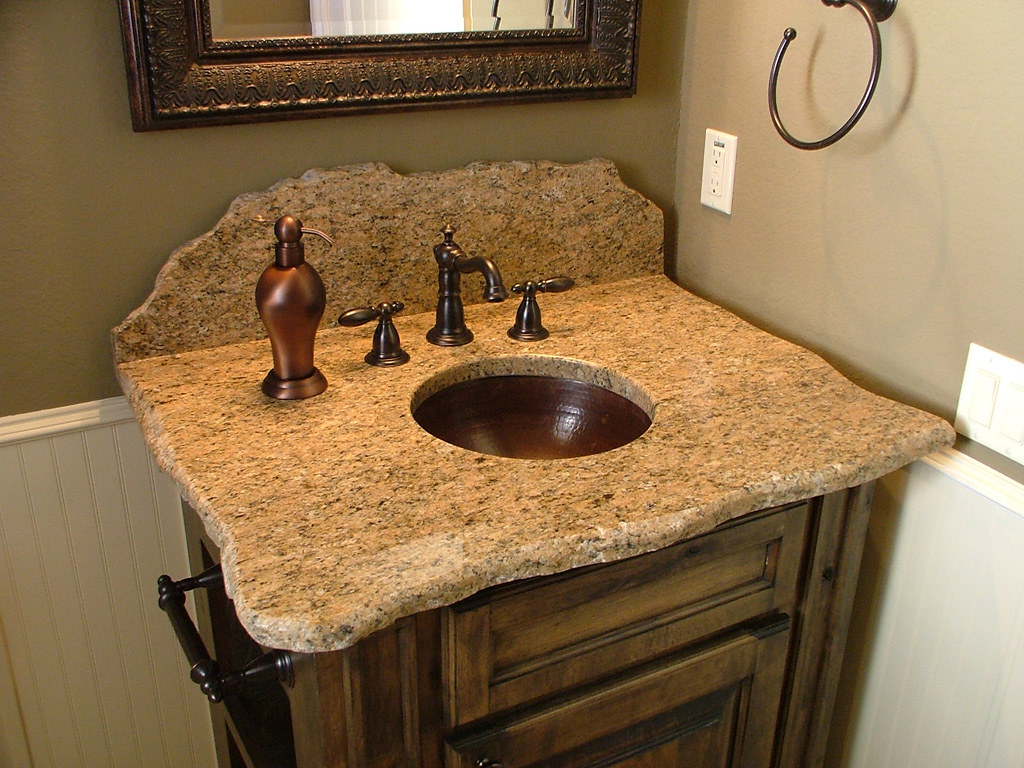This color photograph captures a detailed view of a bathroom, focusing prominently on the sink area. The centerpiece is a distinctive granite sink with an unconventional backsplash that gives the appearance of a broken piece of stone, creating a rugged yet luxurious aesthetic. The sink countertop, made from the same granite, showcases a blend of curvilinear shapes and jagged edges, adding to the rustic charm. This striking granite and copper sink ensemble is mounted on a robust, maple-stained wooden cabinet, which exudes a clunky, rustic vibe.

Adjacent to the sink, a metal bracket is visible, likely serving as a paper towel holder or a hand towel bar. Complementing the sink's design, copper fixtures are used throughout, including a copper-colored liquid soap dispenser that discreetly conceals the brand name, enhancing the bathroom's cohesive look. Above the sink, a towel holder made from a copper-ish or tarnished brass material hangs, featuring an open-ended circular design. This meticulous blend of materials and textures creates a bathroom space that is both rustic and refined.